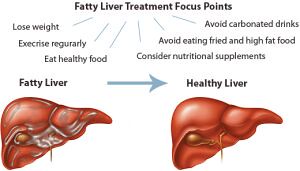The image titled "Fatty Liver Treatment Focus Points" features a detailed comparison between a fatty liver and a healthy liver. The top of the page is labeled with the main focus points for treating a fatty liver. Accompanying the text are two liver images: one marked as "fatty liver" with an arrow pointing towards it, showing a liver with various grayish lumps indicating fat deposits, and the other labeled "healthy liver," displaying a smooth, vibrant red liver. The healthy liver appears more uniform and unblemished.

Under the instructional heading "Fatty Liver Treatment Focus Points," there are several recommendations: 

1. Lose weight
2. Exercise regularly
3. Eat healthy food
4. Avoid carbonated drinks
5. Avoid eating fried and high-fat food
6. Consider nutritional supplements

This chart serves as an educational guide, visually and textually emphasizing the steps to transition from a fatty liver to a healthy liver.